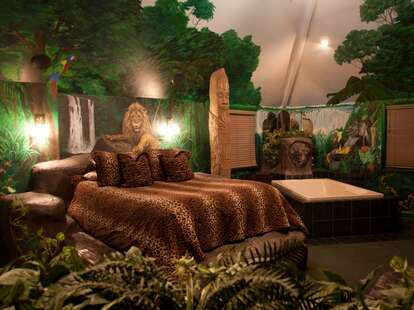The image depicts an intricately themed bedroom with a strong jungle motif. Dominating the center and slightly to the left is a large bed adorned with a brown cheetah print blanket and four matching pillows. Above the bed is a mural that stretches across the back wall, richly painted with a jungle scene featuring multiple trees, leafy green plants, a cascading waterfall, a cliffside, and a vibrant parrot perched on a branch. Adding to the room's wild aesthetic, a regal lion is also part of the mural. To the immediate right of the bed, there is a minimalist white table, and further behind it stands a totem statue. The room is framed by a lush array of green leafy plants that occupy the lower portion of the image, giving the impression of an indoor jungle. The ceiling itself is an extension of the theme, painted to resemble a leafy canopy. The overall color scheme includes browns, greens, tans, whites, yellows, and a touch of red, carefully selected to enhance the jungle atmosphere.